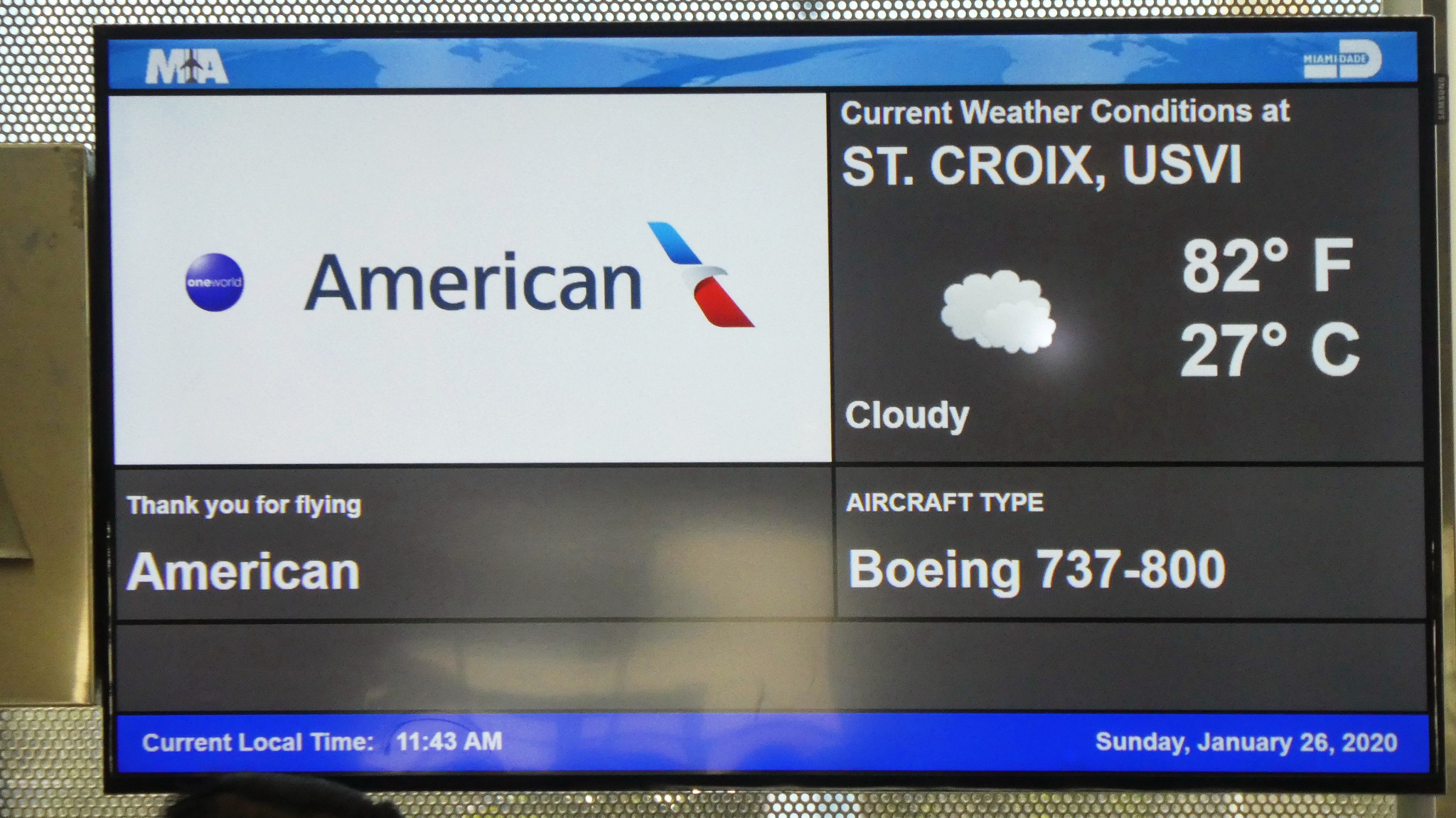The image depicts a digital monitor at an airport boarding gate. At the top of the screen, there's a thin blue strip displaying "MIA" with a black silhouette of an airplane between the letters. Just underneath, on the left side, there's a large, white rectangular box with "American" in black font, accompanied by the American Airlines logo, which features a stylized eagle head with a red stripe below it and a blue stripe above it. 

Adjacent to this, on the right, there's a dark gray box with white text that reads, "Current weather conditions at St. Croix, USVI: 82 degrees Fahrenheit, 27 degrees Celsius. Cloudy," alongside a small icon of a white cloud. 

On the lower part of the screen, the left side features a message in white font saying, "Thank you for flying American," while the right side displays, "Aircraft type: Boeing 737-800." 

At the very bottom, another thin blue strip runs across the screen, with the lower left corner showing, "Current local time: 11:43 a.m.," and the lower right corner indicating, "Sunday, January 26, 2020."